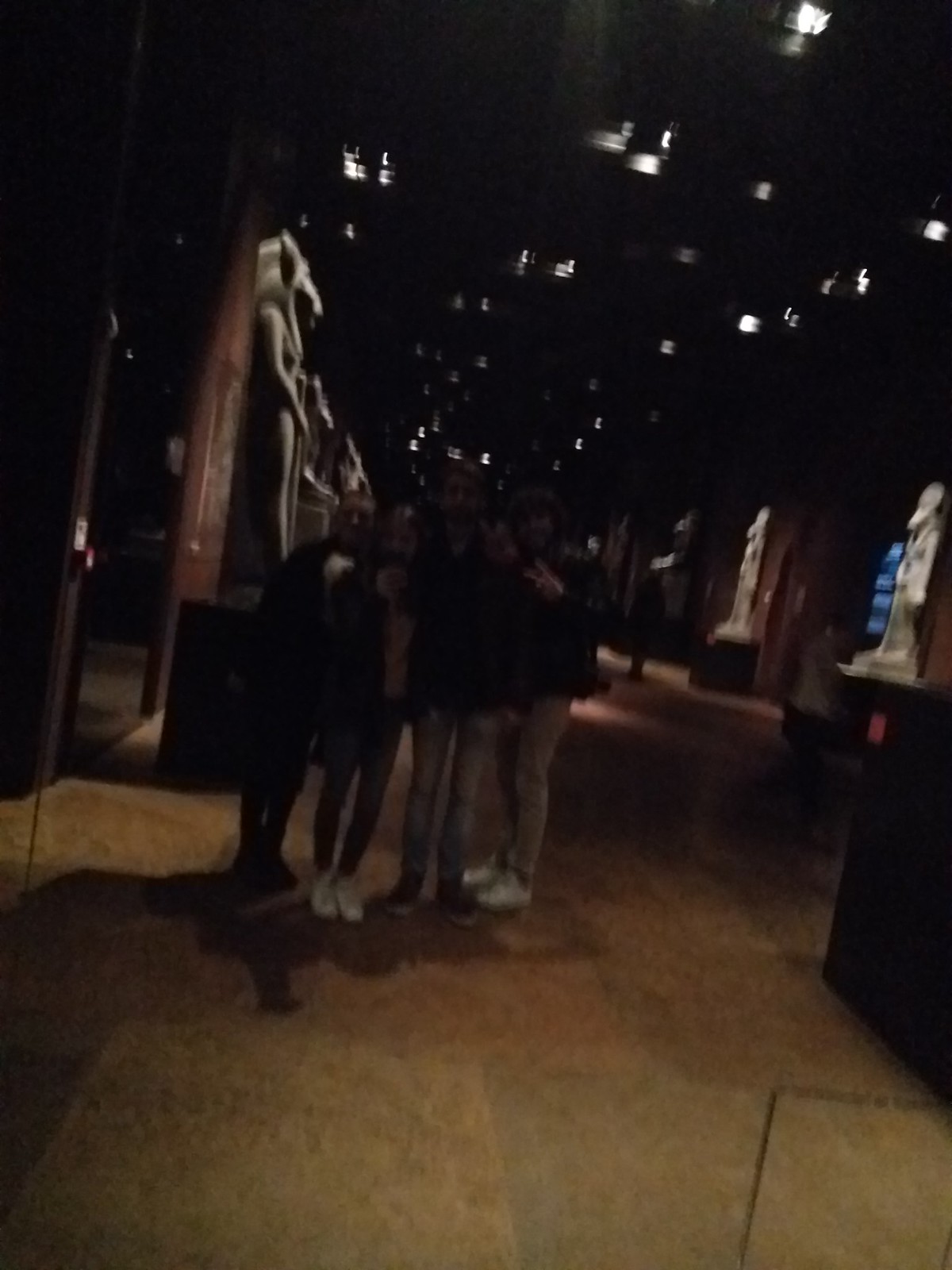The photograph captures a dimly lit museum interior, focusing on a group of four friends posing for the camera. The wooden floor beneath them is light brown, constituting roughly the lower third of the image. On the left side, a large glass door with a silver handle is visible. Moving from left to right, the group consists of a balding man in a black jacket, white pants, and black shoes; a woman with brown hair, wearing a yellow shirt under a jacket, blue jeans, and white shoes; a tall man with dark hair and a possible beard, dressed in a jacket, blue jeans, and brown shoes; and another man with black hair, making a peace sign with his left hand, dressed in a black jacket, blue jeans, and white shoes.

In the background, both sides of the image feature Egyptian-style statues on wooden platforms, each statue bathed in spotlight from the ceiling fixtures, which are scattered across the jet-black ceiling. The statues are grayish in color and arranged three deep on both the left and right sides. Despite the image's low resolution and lack of flash, the statues' details are somewhat distinguishable thanks to the strategic lighting.